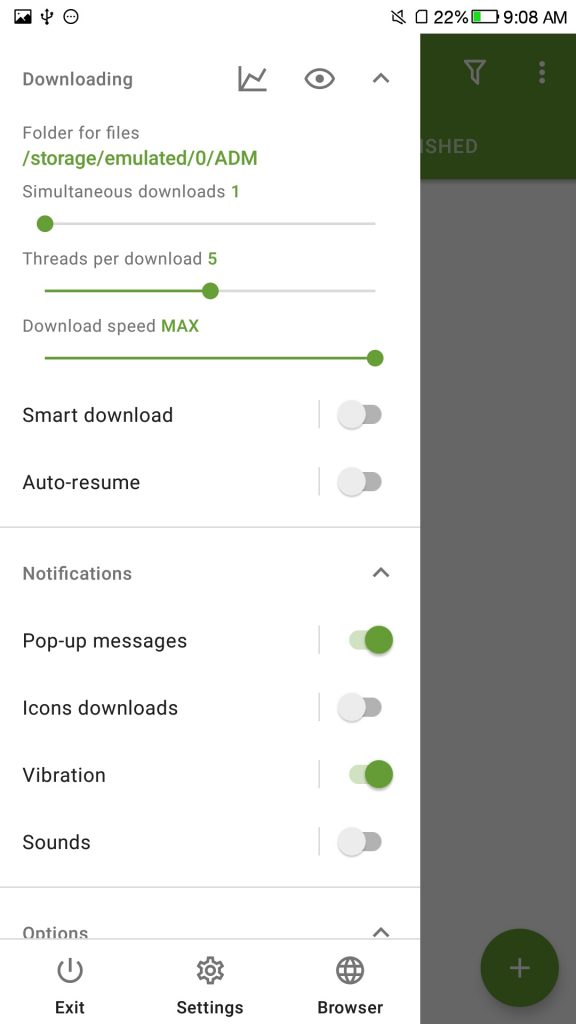This detailed screenshot is captured from a cellphone display. The device shows a battery level of 22% and the time is 9:08 AM. Notification sounds appear to be muted, as indicated by the icons at the top. The main screen background is white, featuring prominent blue and green stripes across the top.

A side menu overlay is present on the screen. At the top of the menu, it reads "Downloading," followed by the path: "folder for files: /storage/emulated/0/ADM." It indicates that one simultaneous download is occurring, controlled by a slider which is positioned all the way to the left. The "Threads per download" option is set to 5, with its corresponding slider placed in the middle. Meanwhile, the "Download speed" is set to "max," indicated by a far-right slider position.

Below these settings, "Smart download" and "Auto resume" options are turned off, whereas "Notifications" for pop-up messages is on. The "Icons" for downloads are off, "Vibration" is on, and "Sounds" is off.

At the bottom of this overlay, there are several options displayed: a drop-down menu labeled "Options," along with "Exit," "Settings," and "Browser" buttons.

Although the app or website in question is not identified by any visible logos, the interface suggests it could be a download manager rather than a job website, given the detailed focus on downloading parameters and settings.